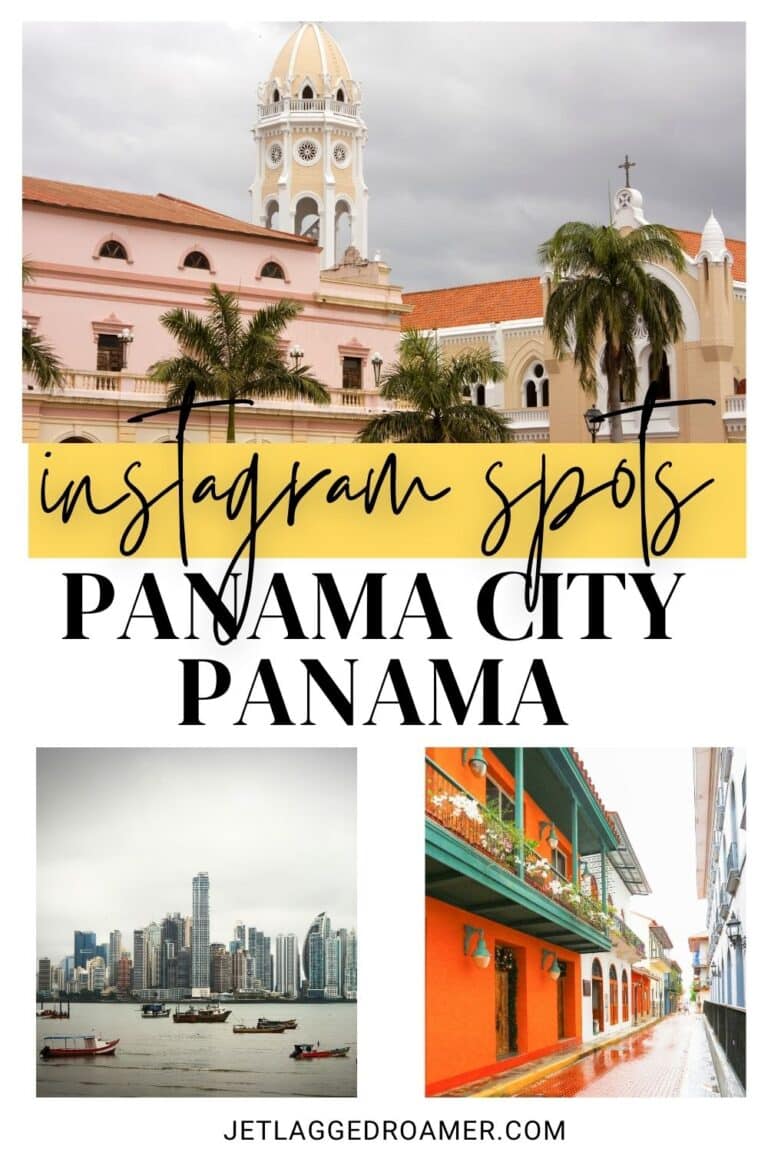This collage features three stunning photographs highlighting picturesque scenes from Panama City, Panama. 

The top image showcases a beautiful light tan beige church adorned with white detailing and crowned by an orange roof. Graceful palm trees decorate the foreground, adding to the tropical charm of the scene. 

Below this image, two banners are displayed: a vibrant yellow one with the words "Instagram Spots" in bold black font, and a white one stating "Panama City, Panama," also in black font.

The photograph on the bottom left presents a breathtaking panoramic view of the city. The skyline is captured from a distance, with numerous boats dotting the serene waters in the foreground, creating a harmonious blend of urban and maritime life.

The bottom right photograph depicts a quiet street, featuring an eye-catching orange building with a green balcony. The street appears slightly wet, hinting at recent rain, while the overcast sky casts a soft, white light over the scene, enhancing its tranquil and serene atmosphere.

The image collage is credited to jetlaggedroamer.com, prominently mentioned at the bottom of the collection.